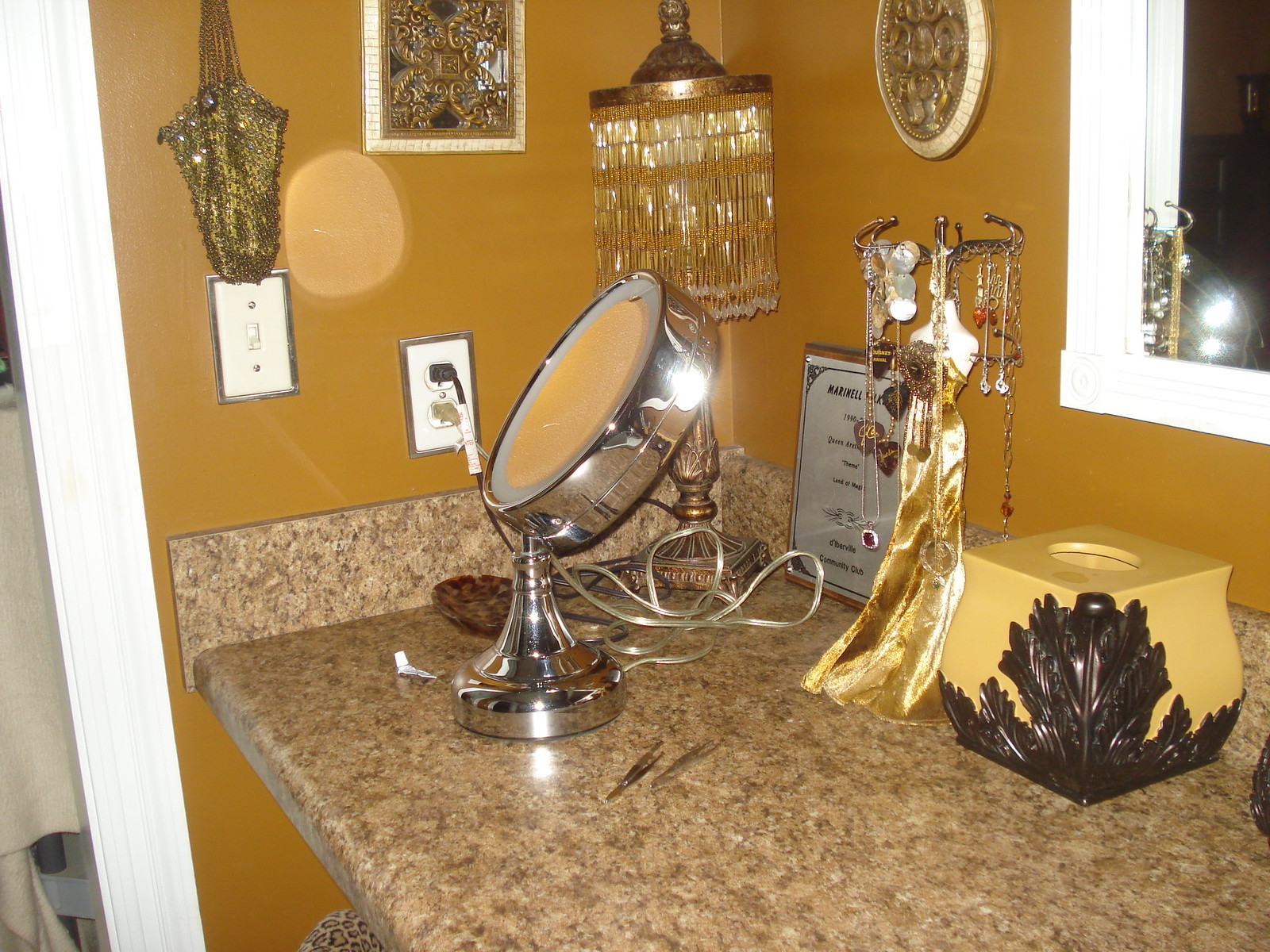The image showcases a countertop area characterized by Formica surface in various shades of brown, accented by a small backsplash along the edge. The surrounding walls are painted a rich, deep gold color. Attached to the wall is a white light switch and a white electrical outlet. Illuminating the space is a lamp with a cylindrical glass shade composed of intricately arranged glass pieces, capped at the top, and supported by a bronze stemmed stand.

On the countertop, there is an elegant sculpture designed for hanging necklaces. Next to it sits a yellow tissue box adorned with a leaf pattern that extends from the bottom towards the top. Mounted on the wall above the countertop is a mirror, reflecting parts of the room's decor. Flanking the mirror are two framed pictures or decorative items, contributing further to the aesthetic appeal of the space.